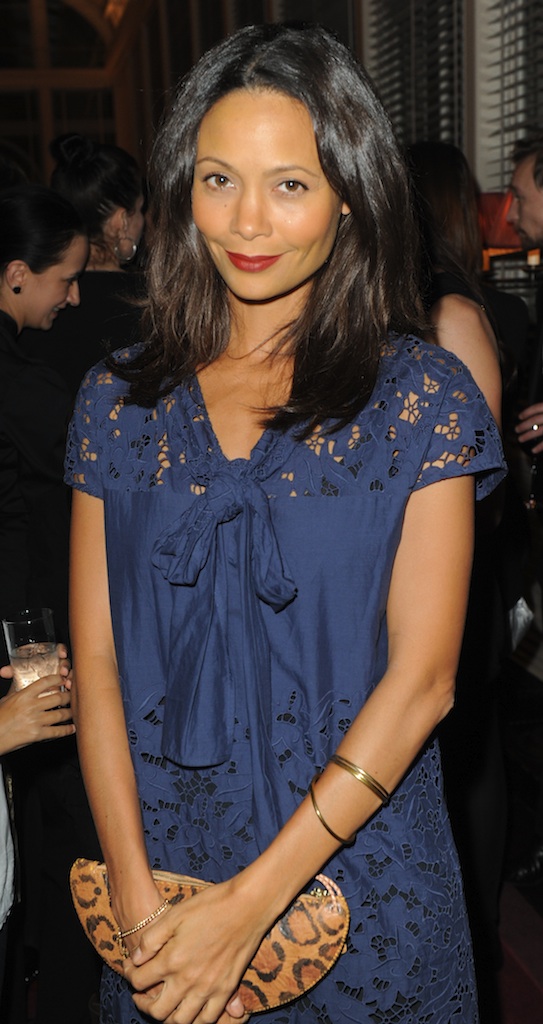The photograph captures a striking image of a woman from her upper legs to the top of her head, with her lower legs cut off by the edge of the frame. She is positioned centrally, facing forward and smiling warmly at the camera. Her outfit is a distinctive blue short sleeve dress with lacy shoulders and a decorative pattern created by holes. A blue tie accents the front of her dress.

In both her hands, which are held at the center of her body, she holds a bean-shaped clutch adorned with a leopard print design and featuring a zipper on top. Adorning both of her wrists are multiple gold bracelets. She has long, dark brown or black hair and is wearing striking red lipstick.

The background reveals a lively scene where multiple people are mingling, holding drinks, and engaging in conversation, suggesting that the setting might be a party or social gathering. Blurred figures in mostly dark attire contribute to the atmosphere, with a notable presence of black blinds covering multiple windows on the far back wall. Additionally, over her right shoulder are more people, and to her left, a person holding a glass of liquid can be seen in the frame.